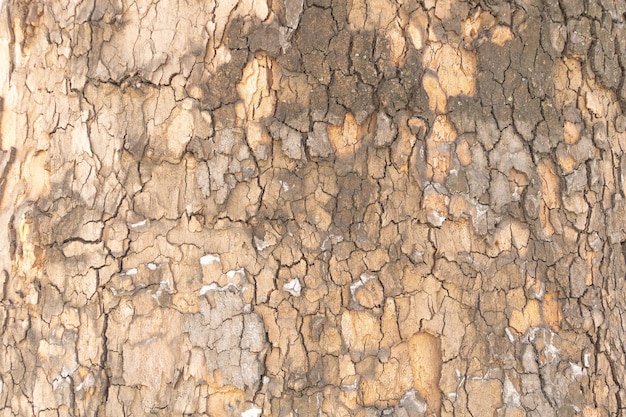This image is a close-up of the trunk of an old, possibly very large tree, showcasing its intricate bark. The bark displays a cracked and scaled appearance, reminiscent of a serpent's skin. The colors range from a lighter tan wood with some areas of muted gray to distressed darker grayish-brown patches that look wet. Medium brown tones can also be seen, especially in the bottom corners where shadows create a deeper contrast. Some of the bark is peeling off, revealing the different shades of beige and the perforated texture as each small piece gradually detaches. There's no additional background, objects, or text in the image, focusing solely on the tree's textured surface.